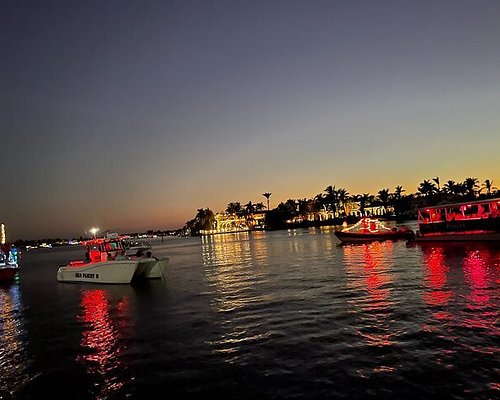The photograph depicts a serene waterscape during the twilight hours, where the sky transitions from an orange-yellow near the horizon to various shades of blue and dark blue as it ascends. The main focus is the dark, rippled water, reflecting lights from scattered boats and buildings in the background. The horizon features a shoreline lined with palm trees and brightly lit houses, including a prominent mansion or elaborate structure. Several boats, including two on the left heading in one direction and two on the right going the opposite way, navigate the waters. Enhanced with red, yellow, and blue lights, the scene is picturesque with the setting sun casting a warm glow over the landscape.